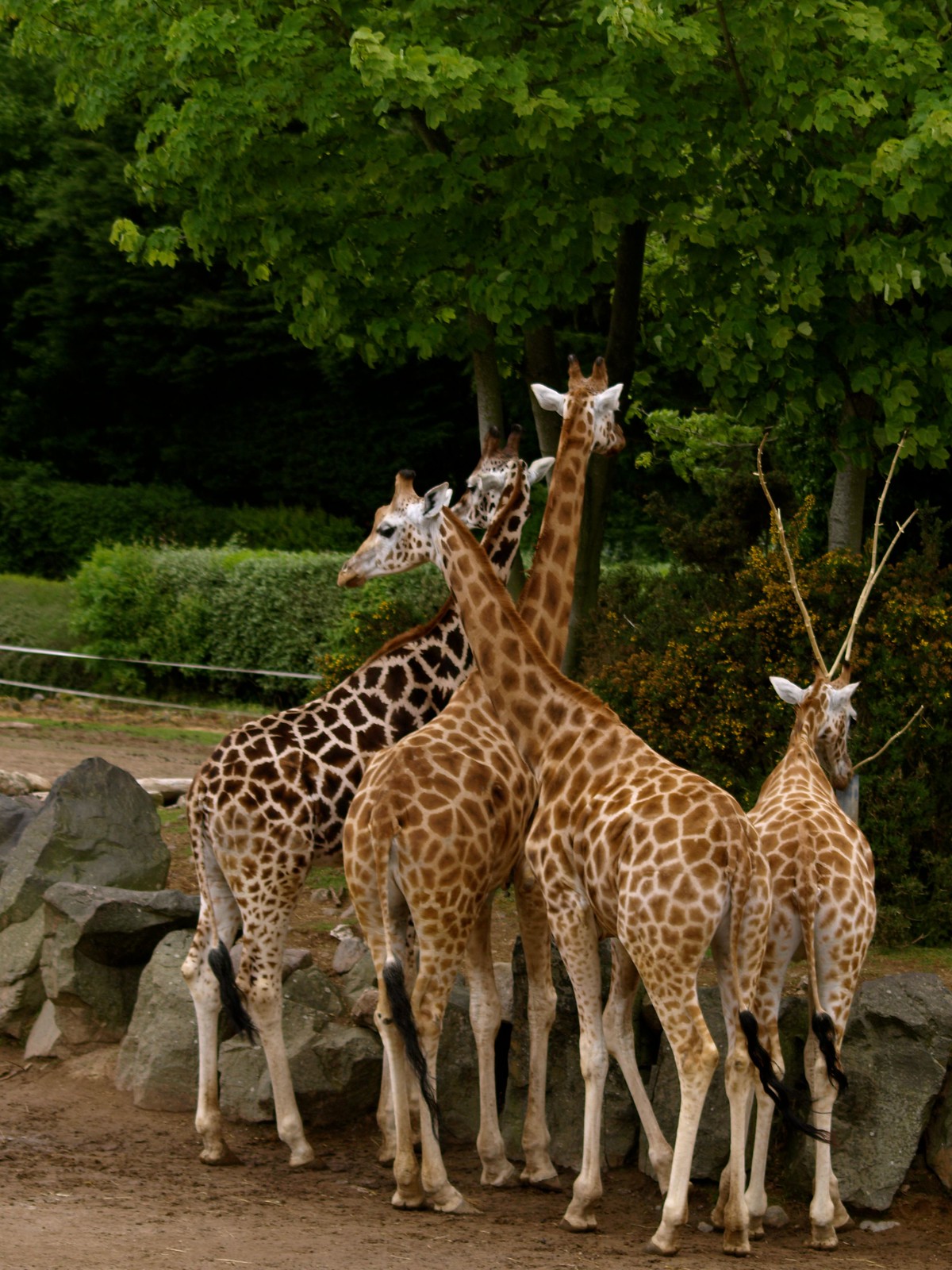In this color photo taken at a zoo, four giraffes are seen standing on packed dirt in front of a line of giant boulders that appear to form part of their enclosure. The giraffes have long necks and distinctive patterns on their skin. Three of them, all with lighter brown and cream coloring, face away from the camera, showing their long tails with black tips. The fourth giraffe, positioned on the far left, has a noticeably darker brown pattern and seems to glance off to the left. In the foreground, one can see a leafless tree, and in the background, lush green shrubs and tall leafy trees add a burst of color to the scene. There is no sky visible, and no people are present in the photo, emphasizing the natural, serene environment of the animal enclosure.